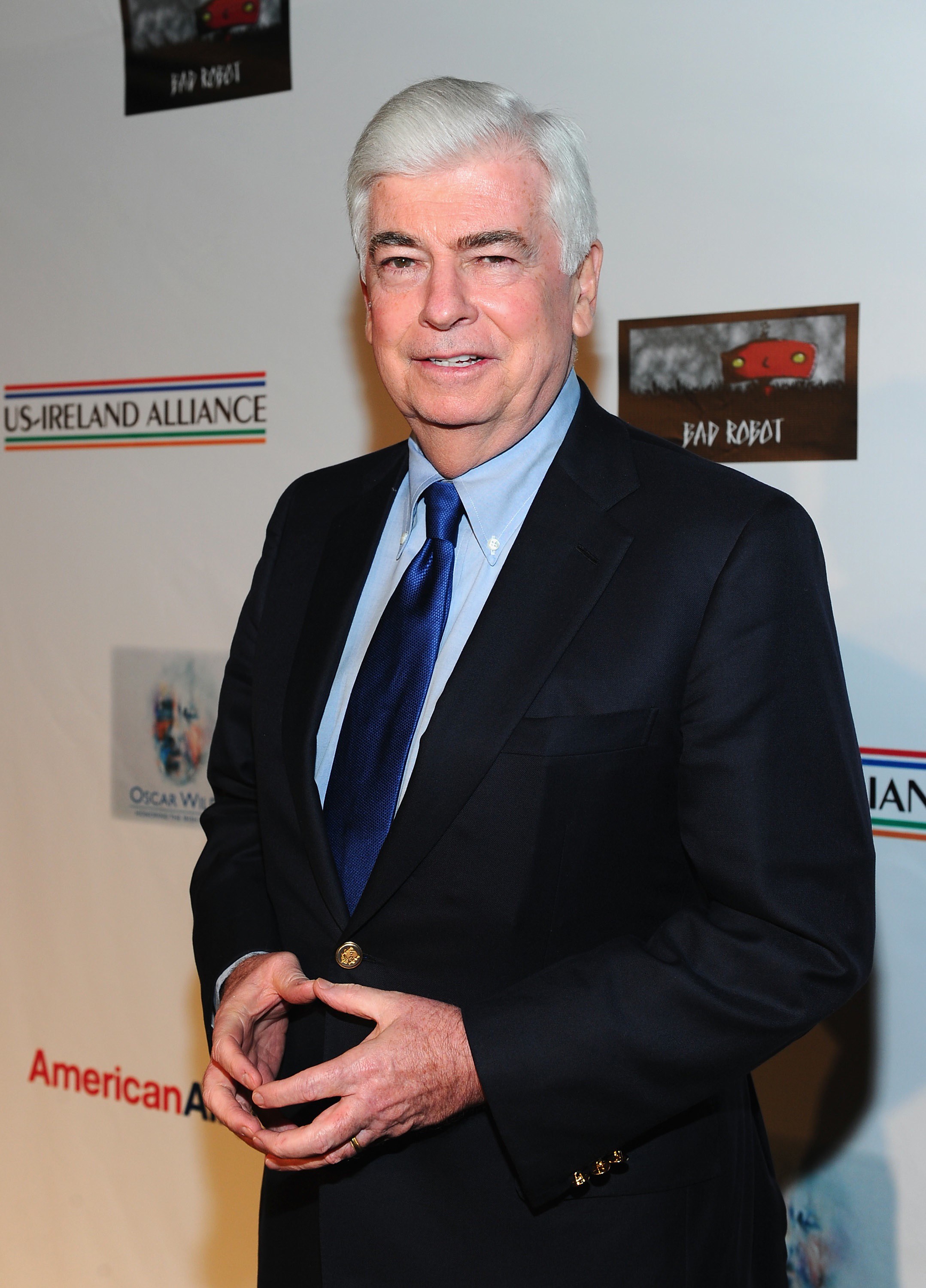In the image, an older gentleman, potentially an actor, director, or writer, poses with a composed yet subtly cheerful expression, his short white hair neatly combed over. He wears a dark suit, possibly navy or black, complemented by a light blue button-up shirt and a satin blue tie. His hands are positioned at mid-torso, fingers interlaced to form an 'O' shape. To the left of him is the recognizable logo for Bad Robot, a well-known film and television production company. The backdrop features a step-and-repeat banner adorned with logos, including those of American Airlines and the US-Ireland Alliance, while some other logos remain partially obscured.